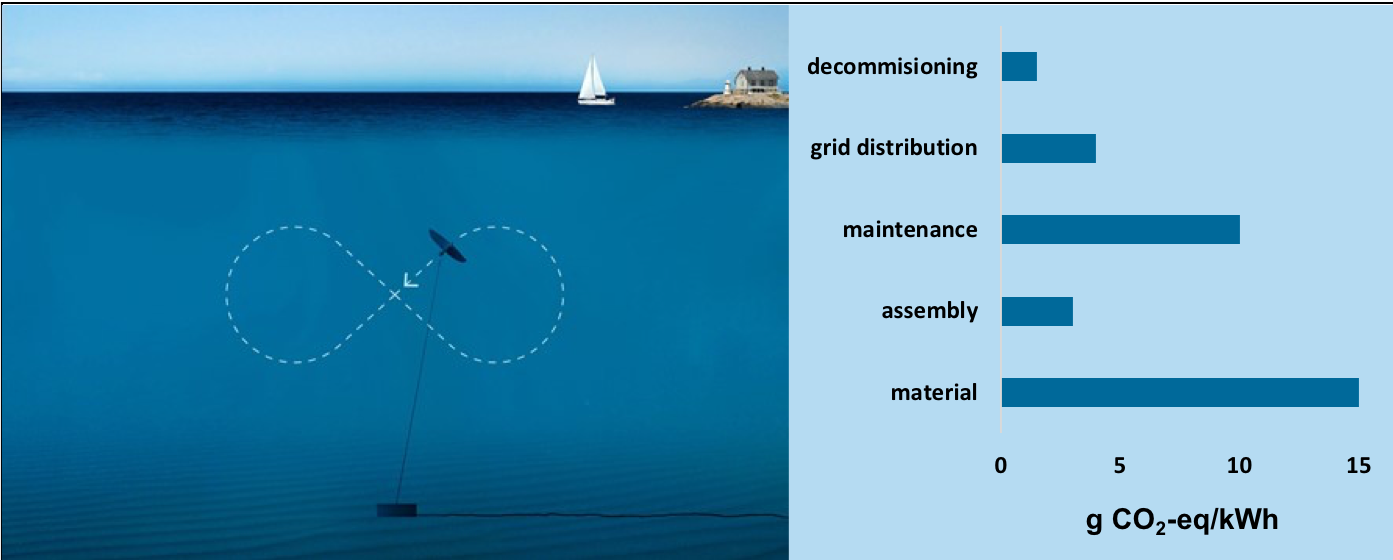The image is a detailed scientific diagram primarily featuring an underwater scene with a large body of water. Central to the diagram is a figure-eight dashed line, suggesting some path or current, being followed by a bird. Above the water, in the distant background, there's a small sailboat and a tiny island with a house on it. The right side of the diagram includes a graph with an x-axis ranging from zero to fifteen and a y-axis labeled with terms such as decommissioning, grid distribution, maintenance, assembly, and material. At the bottom of the graph, there's a formula labeled as GCO2-EQ-KWH, likely measuring grams of carbon dioxide equivalents per kilowatt-hour. The entire image uses various shades of blue, with black text, aiming to convey information related to CO2 emissions and possibly the environmental impact of maritime activities.